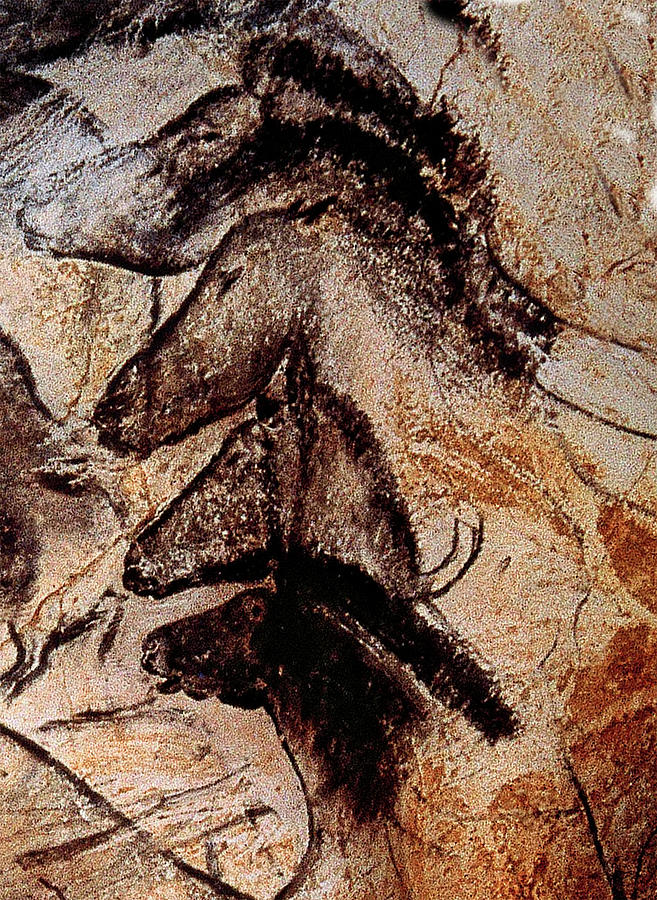The image depicts cave drawings on a textured red sandstone wall, featuring four stylized and somewhat rudimentary horses progressing vertically down the surface. Each horse's head extends from an elongated neck, with the horses stacked one above the other. The horses appear to be drawn with a dark substance, possibly charcoal, with variations in shading and detail among them. The top horse showcases a more prominent dark mane, while the others gradually diminish in both detail and color intensity. The bottom horse is the most richly colored, in dark brown, while the others show less coloration and detail, suggesting different ages or stages of artistic completion. Despite a lack of intricate features like nostrils or mouths, the general form and position of the horses are clear under the direct illuminating light. The background is marked with additional vague lines that could suggest other horse figures or simply be part of the wall's natural texture. The picture is captured in high resolution, making all elements sharply visible, though the geographic location of the cave remains unspecified.